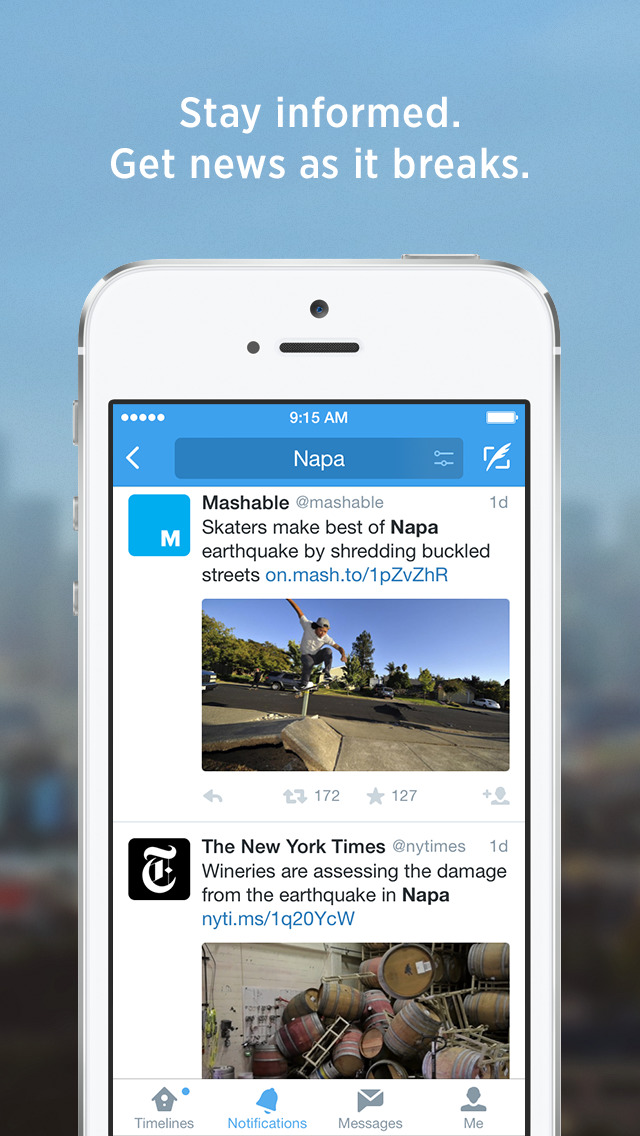Caption: 

A blurry image predominantly featuring a sleek white smartphone with silver edges. The top of the image displays the word "Texas," followed by the phrase "staying forward," suggesting perseverance or optimism. The screen of the smartphone includes several small details, such as "915," possibly indicating a time, and a full battery icon. Notably, there are mentions of a blue square and the word "mashable" alongside "unmashable," hinting at digital content. Additionally, the text references "1D Scars" and "best of Napa," likely pointing towards an article or story about overcoming adversity in Napa after an earthquake, with further information to be found on a provided URL.